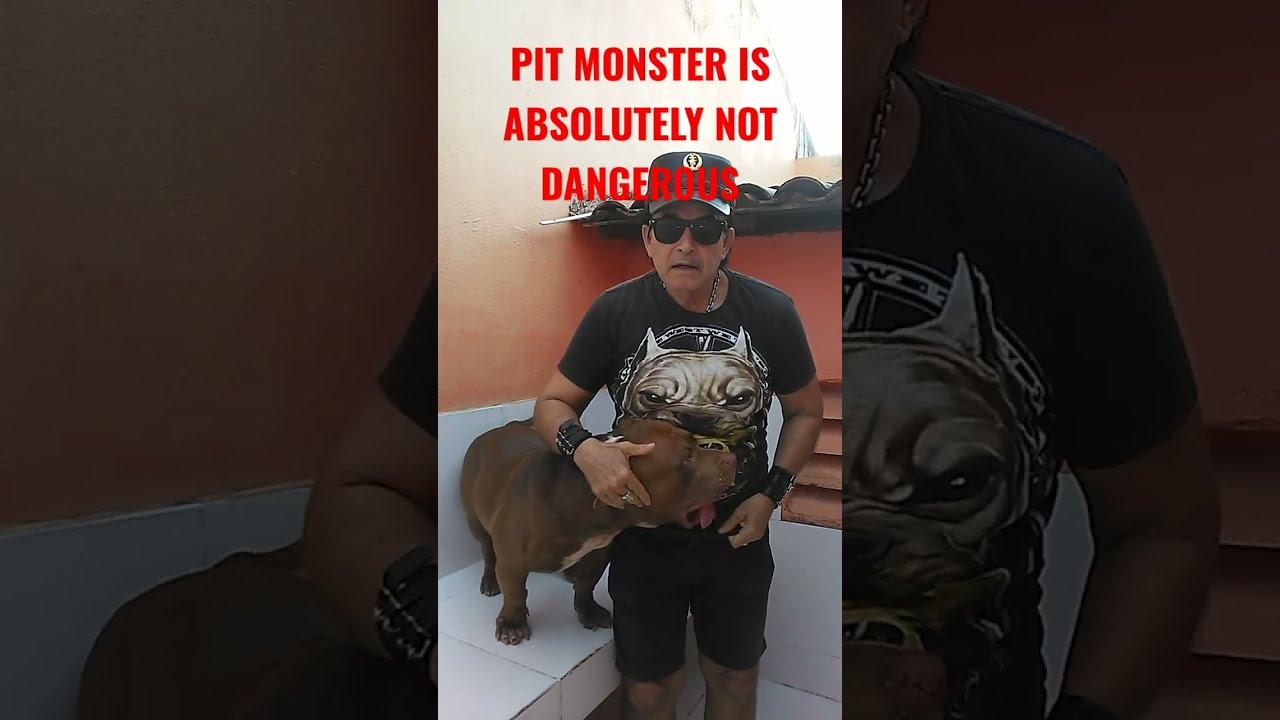The image is a three-panel composition with the central panel displaying a vivid photograph of a man and his dog, accompanied by darker, zoomed-in versions of this central image on the left and right sides. The central picture features a man dressed entirely in black, with a black cap, sunglasses, t-shirt, and shorts. His t-shirt displays a large image of a bulldog's head. The man has black wristbands adorned with metal studs and a silver chain around his neck, and he is posed with his arm around a brown pitbull with a white blaze on its chest, whose face is turned towards the man's abdomen. The dog is standing on a white bench beside the man against an orange-peach concrete wall and a corrugated roof overhang. At the top of the image, a bold, red, all-caps text reads, "PIT MONSTER IS ABSOLUTELY NOT DANGEROUS." The left and right panels, slightly darkened and zoomed in, partially reveal the man's arm and the dog's body, as well as parts of the shirt, arm, head, and wall background.